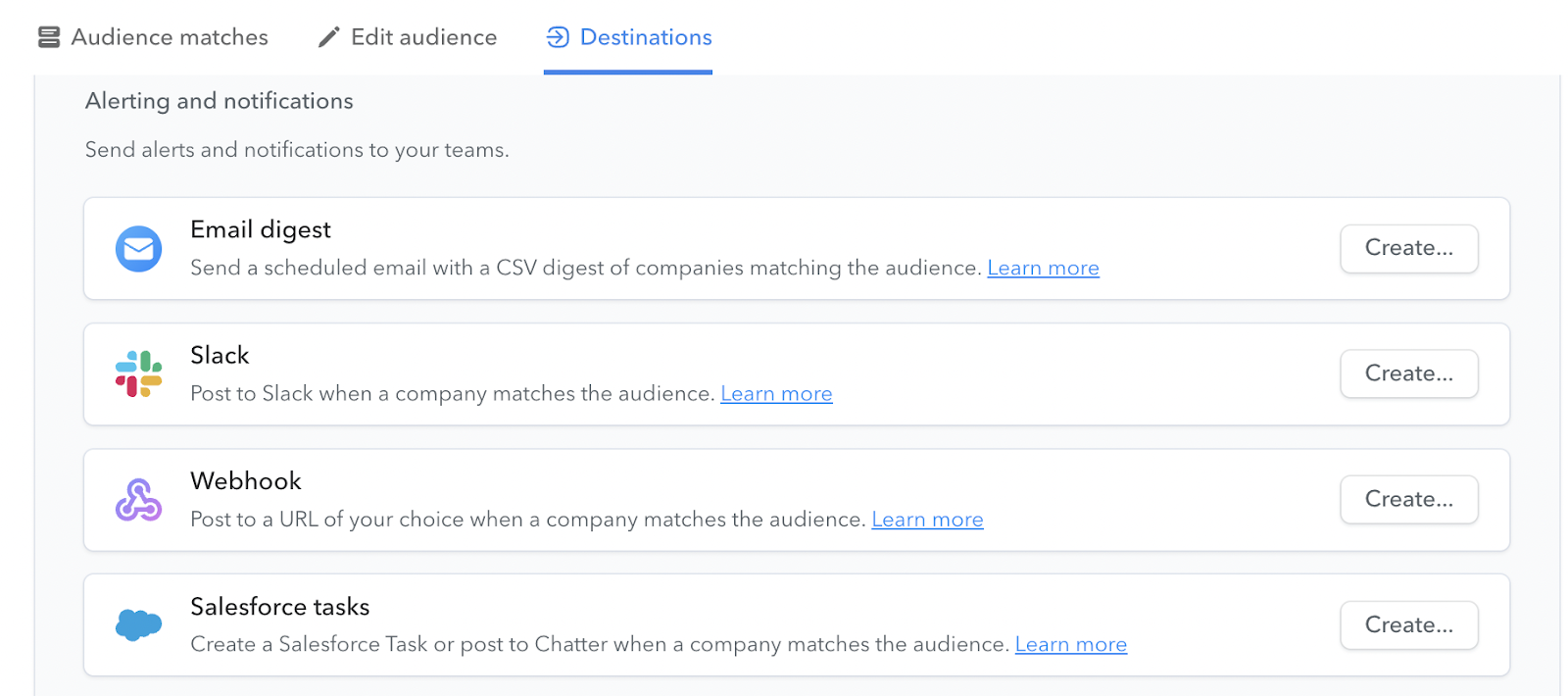The image titled "Audience Matches" prominently features several interface elements related to alerting and notifications. At the top, there is a crayon icon accompanied by the text "Edit Audience." Adjacent to it, the word "Destinations" is displayed in blue with a corresponding blue arrow pointing to the right, underlined in blue for emphasis.

Beneath this header, there is a prominent light gray box labeled "Alerting and Notifications," with the accompanying description, "Send Alerts and Notifications to your teams."

Inside this light gray box are several white cards detailing various notification options:

1. **Email Digest**:
   - Description: "Send a scheduled email with a CSV digest of companies matching the audience."
   - Additional Info: An underlined "Learn more" link.
   - Action Button: "Create" button on the right.

2. **Slack**:
   - Icon: A multi-colored icon featuring blue, gold, and red.
   - Description: "Post to Slack when a company matches the audience."
   - Additional Info: An underlined "Learn more" link in blue.
   - Action Button: "Create" button on the right.

3. **Webhook**:
   - Icon: A purple image.
   - Description: "Post to URL of your choice when a company matches the audience."
   - Additional Info: An underlined "Learn more" link in blue.
   - Action Button: "Create" button on the right.

4. **Salesforce Tasks**:
   - Icon: A blue cloud.
   - Description: "Create a Salesforce Task or Post to Chatter when a company matches the audience."
   - Additional Info: An underlined "Learn more" link in blue.
   - Action Button: "Create" button on the right.

This organized layout provides a comprehensive and user-friendly interface for managing various audience notification methods.